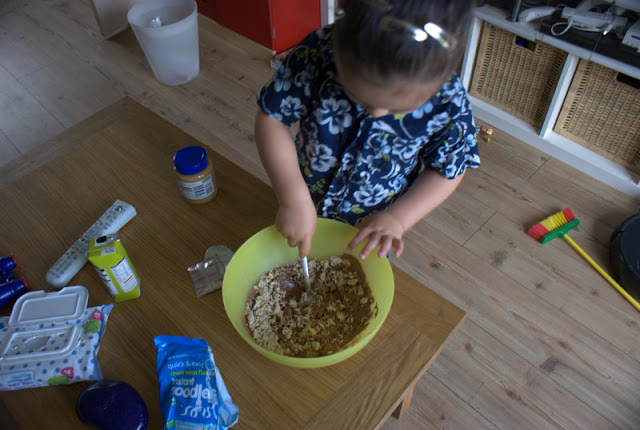In the image, a child is seen wearing a dark blue and white flower-patterned shirt. The child has small, silver metal hair clips adorning the top of their head. They are standing on a light brown floor beside a slightly darker brown table. In front of the child, there is a yellow plastic bowl containing a brown mixture that they appear to be stirring. To the right of the bowl is a jar of peanut butter with a blue lid and a clear plastic body with a white label, filled with a brown substance. A white electrical converter is placed just in front of the peanut butter jar.

In the background, there are white shelves holding brown bamboo baskets with square handles. To the left of the child, there's a white wall and a white basket. A yellow broom with red and yellow bristles lies nearby. Also visible is a lime green box or container with a blue lid, a gray plastic piece to the left of the child, and a blue packet labeled "instant noodles" in white letters. Next to the packet, there's a blue and white polka-dotted bag with a square plastic lid. The setting appears to be a domestic environment with a variety of household items scattered around.